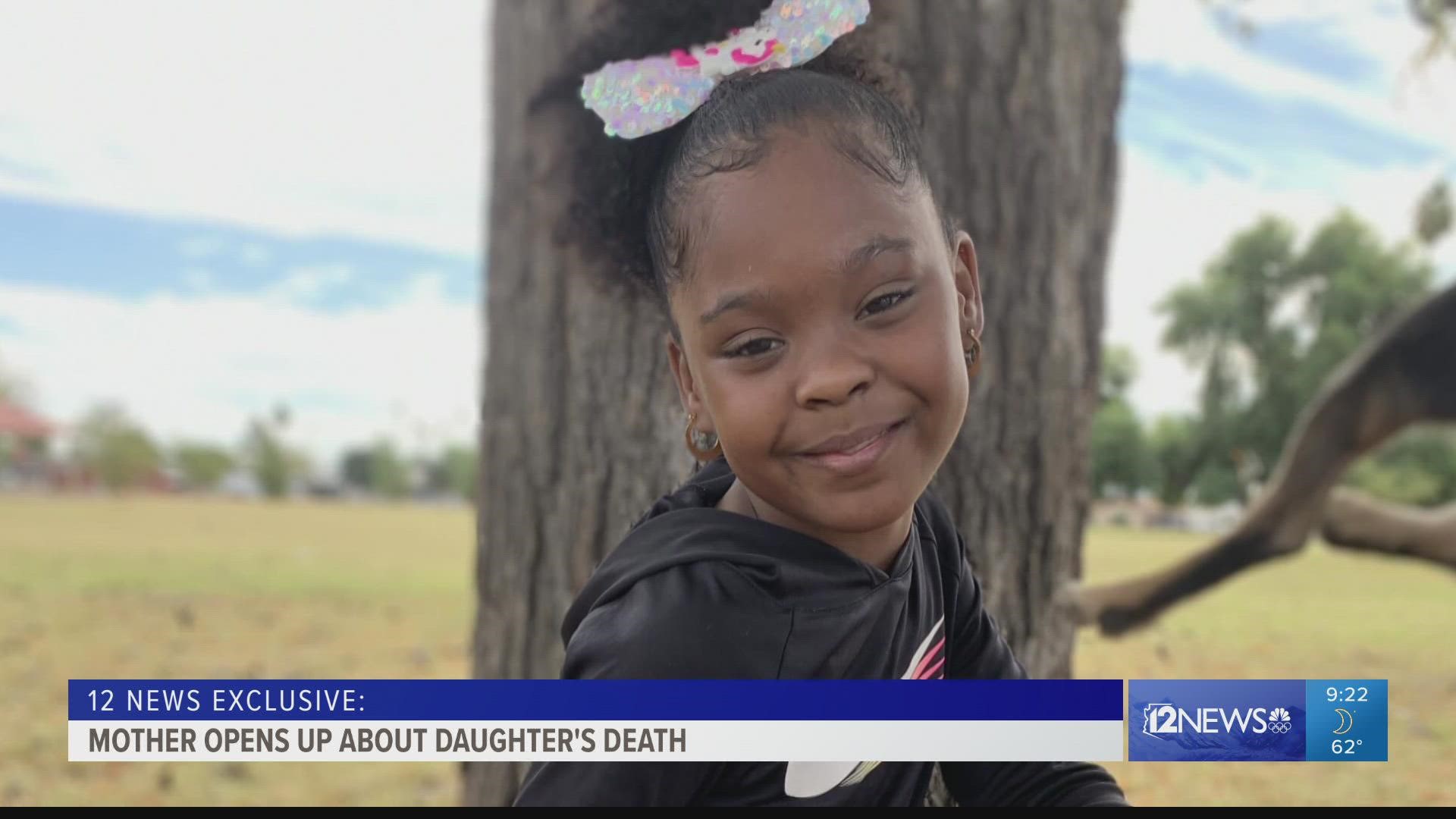The image is a still from a Channel 12 News broadcast featuring the story titled "Mother Opens Up About Daughter's Death." It showcases a young African-American girl standing in front of a tree in a park on a beautiful, partly cloudy day. The girl, donned in a silky black shirt, has her hair styled in a ponytail adorned with a white and glittery bow. Her expressive, lovely smile is directed slightly downwards at the camera. Behind her, the park's blurred background highlights yellowish ground and additional trees. At the bottom of the screen, a blue and white news ticker reads, "12 News Exclusive. Mother Opens Up About Daughter's Death," with the Channel 12 News logo, the time "9:22," a moon icon, and the temperature "62 degrees" displayed next to it.